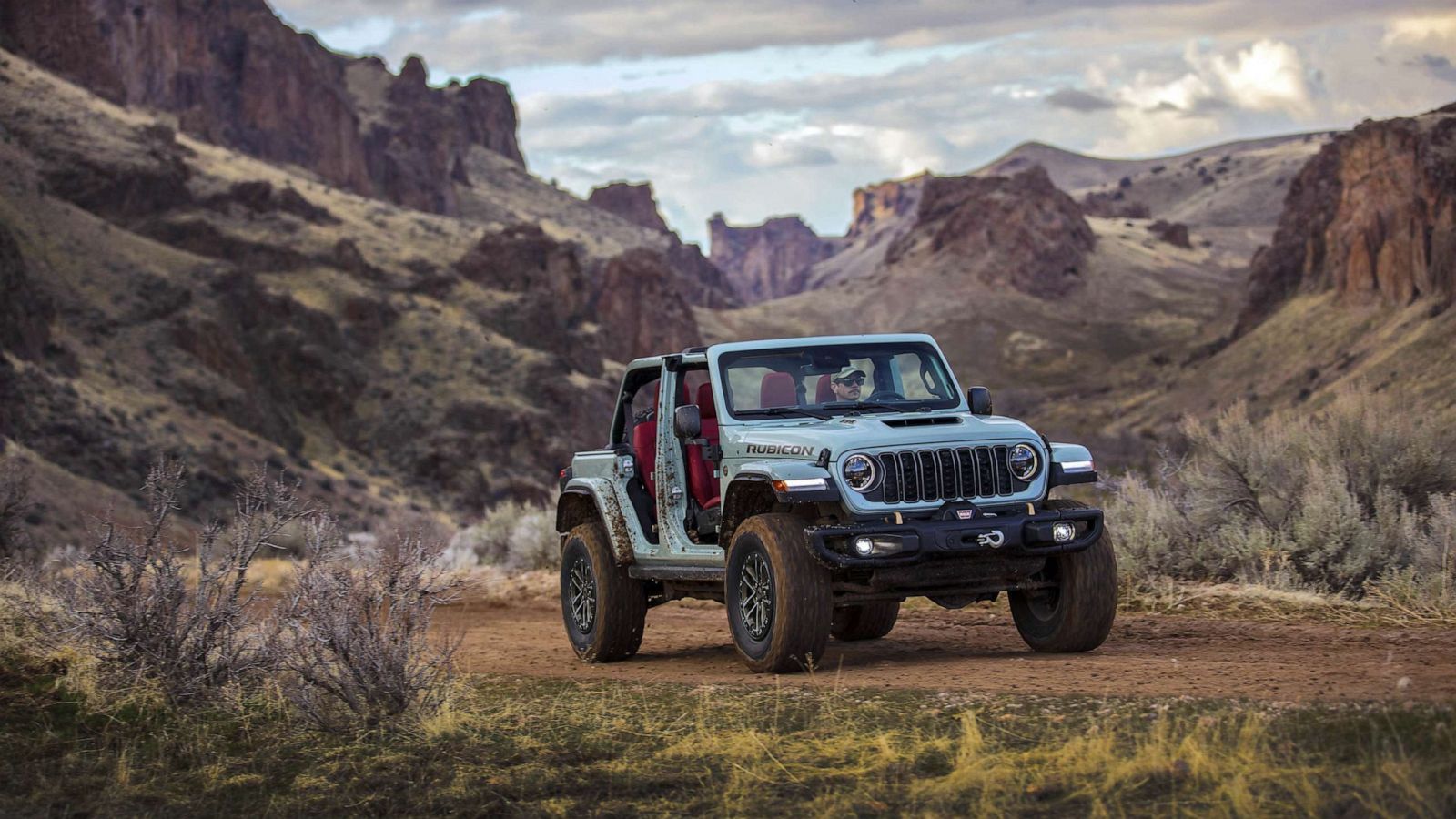The image showcases a rugged, light blue Jeep Rubicon with no doors or top, parked in a desert canyon or possibly in a realistic museum exhibit. Mud-covered, tall tires emphasize its off-road capability. A light-skinned man, sporting a baseball cap and dark sunglasses, is behind the wheel. The Jeep features a red interior, adding a splash of color. The backdrop features high, rocky mountains tapering downwards with crispy, dry plant life, giving the scene a wide open, arid feel. The sky above is partially cloudy, casting a light gray-blue tint over the landscape, creating a dramatic, overcast ambiance. The blending of realistic elements and potential mural-like qualities of the backdrop suggests this could be an advertisement or display.